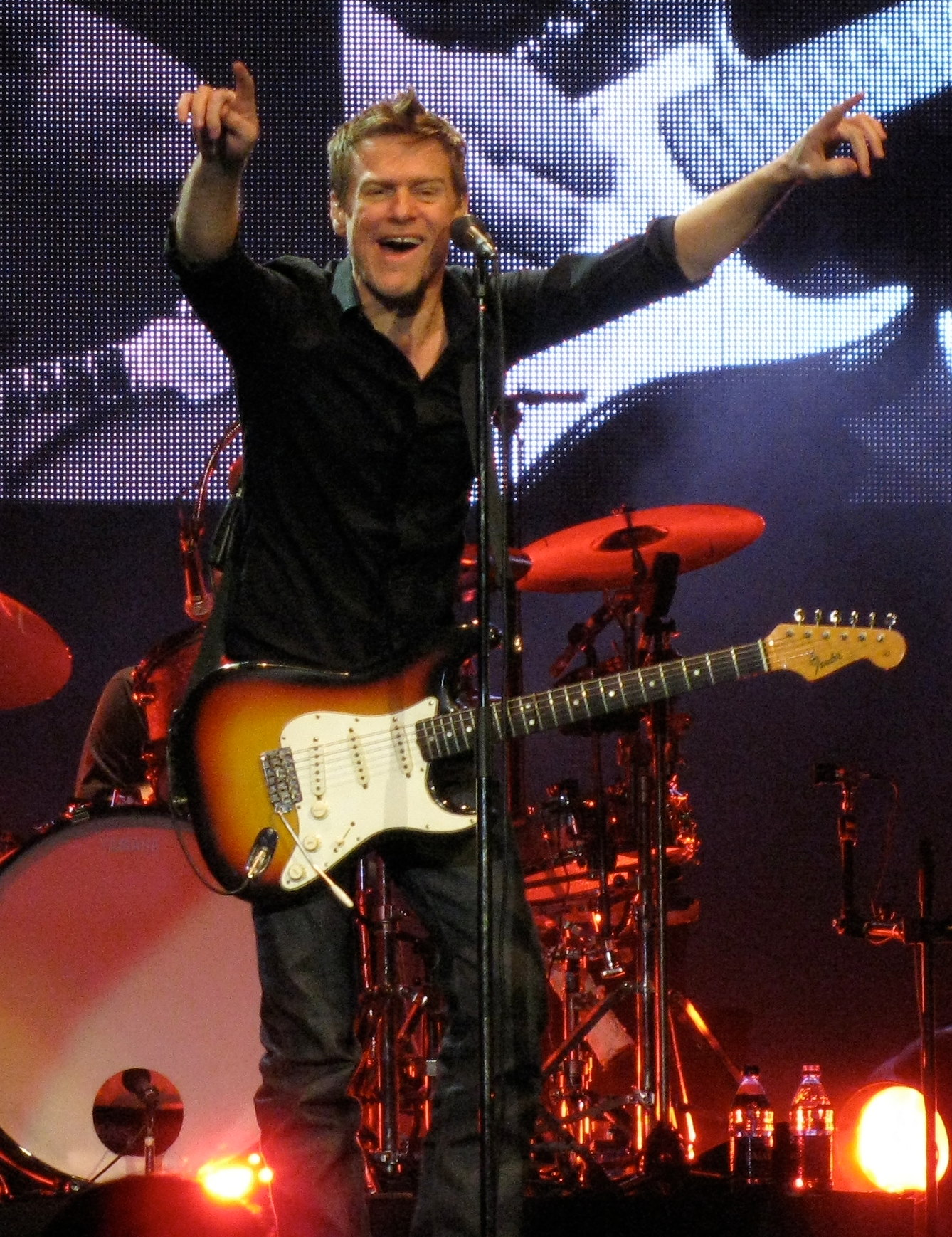The photograph captures an electrifying moment at a concert with a central focus on a dynamic singer-guitarist. Dressed in a black button-up shirt with sleeves rolled halfway and black jeans, the artist, who has light skin and spiky light brown hair, exudes energy. He stands at the center of the stage, his mouth open in a spirited exclamation or song, smiling and pointing both arms towards the audience with fingers upraised. His guitar, a striking blend of orange, black, and white, hangs from a strap around his neck. Positioned before him is a completely black microphone on a stand.

In the background, a drum set is partially visible, predominantly the cymbals, as the drummer is mostly obscured by the frontman. The stage is bathed in light, with orange highlights illuminating the drum set. Further enhancing the scene, an LED screen projects a black and white image which seems to amplify the concert experience for the audience. This screen displays a close-up of a guitar and possibly another guitarist playing. Additional stage details include water bottles on the floor and ambient red lighting complementing the overall vivid atmosphere of the performance.